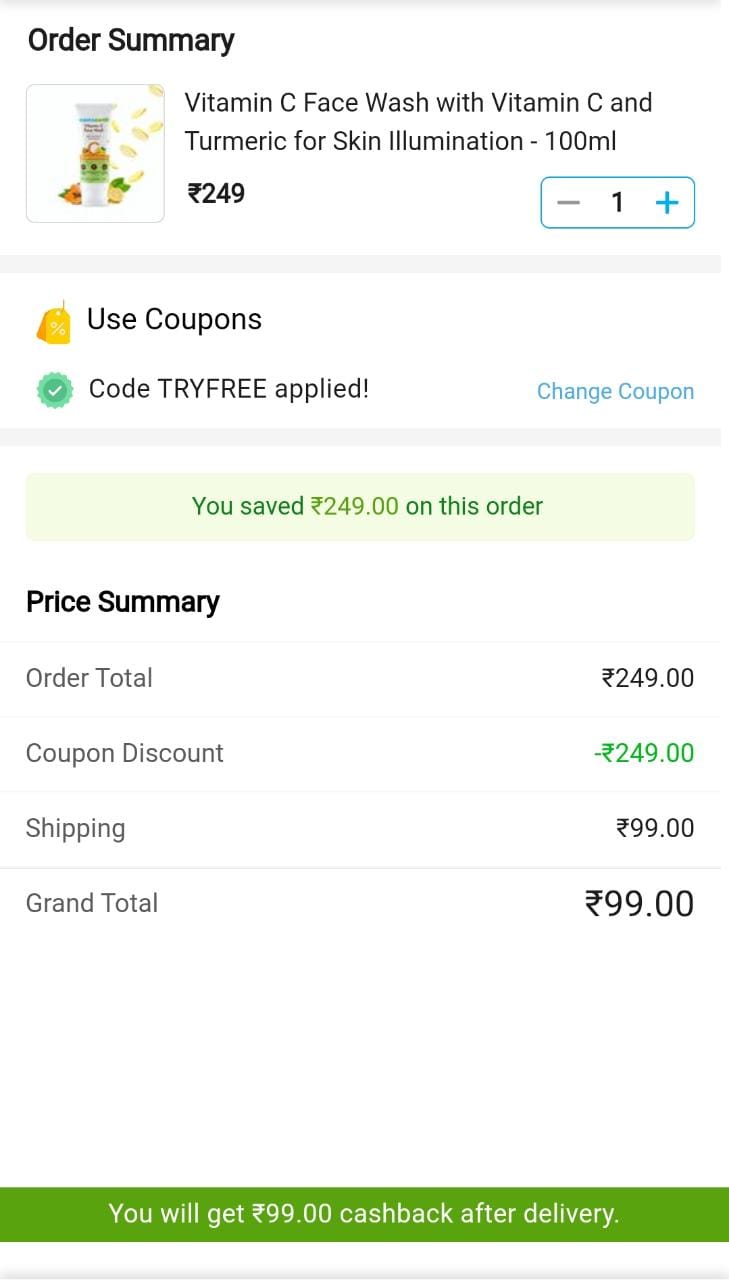The image depicts an "Order Summary" titled in black font at the top. Below the title, there is a detailed listing of a face wash product described as "Vitamin C Face Wash with Vitamin C and Turmeric for Skin Illumination, 100 ml." The product is presented in a white tube adorned with green designs, along with additional orange and blue accents, and black polka dots on the packaging. Below the product, there is an indication of "1 item in cart."

Further down, there is a section labeled "Use Coupons," featuring a yellow tag icon with a percent sign. The text mentions "Cold Try Free Applied," accompanied by a checkmark within a green circle. In blue font, there is an option to "Change Coupon." The message also indicates a saving of $249 on the order.

The "Price Summary" at the bottom shows:
- Order Total: $249
- Coupon Discount: -$249
- Shipping: $99
- Grand Total: $99

Lastly, there is a green rectangular bar at the bottom stating that the customer will receive "$99 Cash Back after Delivery."